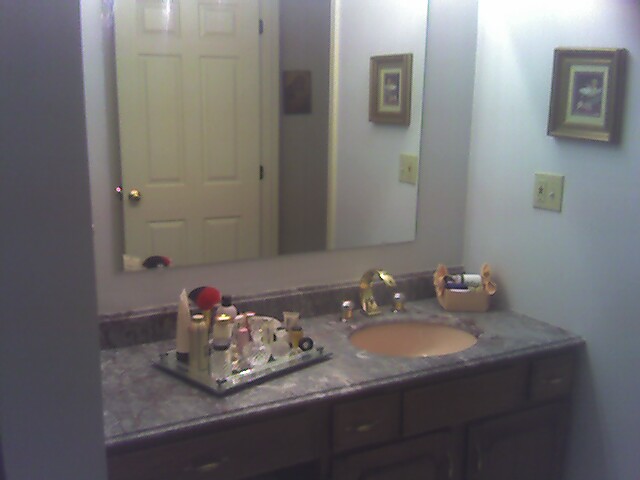In this image, we observe a detailed bathroom setting. At the bottom, there are dark brown drawers positioned directly below a gray countertop. The drawers are laid out from a front-view angle: on the left, there is a longer rectangular drawer followed by a smaller square-shaped drawer, another rectangular one, and finally another small square-shaped drawer. The bottom two drawers are partially visible and are vertically square, making them larger compared to the four horizontal upper drawers.

Above these drawers lies a gray countertop featuring a circular sink. To the right of the sink, there is a tray containing various makeup, hair products, or skincare items, all neatly arranged within a light gray, square-based frame and standing vertically. The faucet, positioned to the right of the tray, is a golden metallic color with gray handles on either side.

Further right, there is a decorative object placed on the countertop. Moving to the wall, the light gray surface hosts a tan square light switch with a dark brown picture frame above it. To the left of the picture, there is a square mirror reflecting a door and part of the wall. On the far left of the image, a portion of the light gray wall is also visible, providing a cohesive backdrop to the bathroom scene.